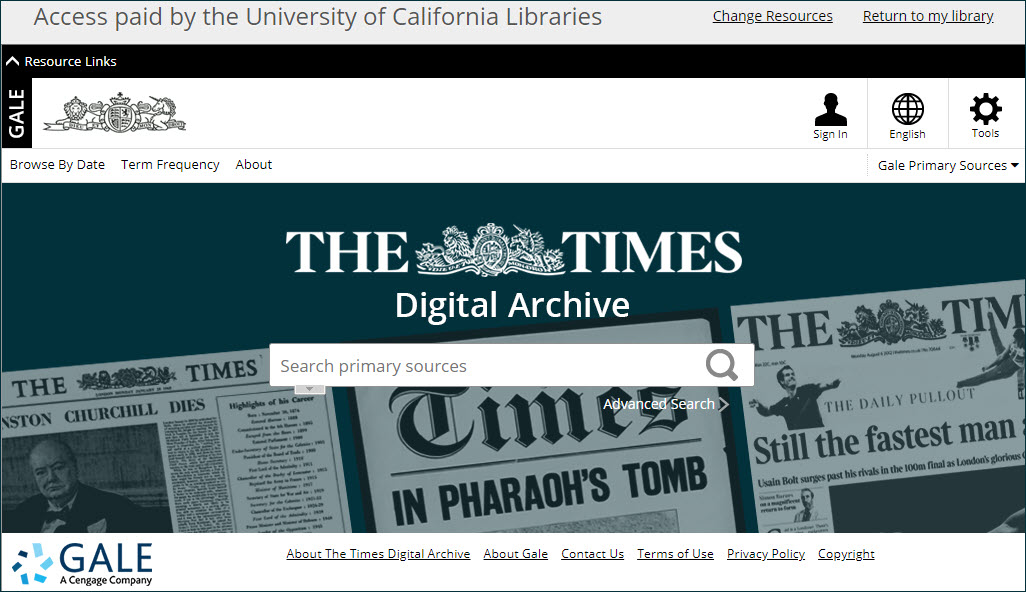The UI displayed represents the Times' digital archive page, marked by distinct features and segments:

1. **Top Gray Bar**: At the top, a gray bar contains the text "Access paid by the University of California libraries" in a dark gray font. Flanking this text are two links: "Change Resources" and "Return to My Library."

2. **Black Side Bar**: Adjacent to the left, there is a vertical black bar featuring an upwards arrow labeled "Resource Links." Along this side bar, the word "Gale" is spelled out vertically, with the letters G, A, L, and E stacked from bottom to top, each letter facing to the right.

3. **Header Row**: The header section includes:
    - **Times Icon**: Positioned to the left, the icon resembles a unicorn intertwined with elaborate scrollwork.
    - **Sign-In Button**: Situated on the right, followed by a vertical gray line, a globe icon next to the word "English," a gear icon beside "Tools," and another faint vertical gray line.
    - **Menu Options**: Following are three primary menu options: "Browse by Date," "Term Frequency," and "About." Then another vertical line concludes this section.

4. **Gale Section**: Towards the middle, below another vertical separator, is the "Gale Primary Sources" dropdown menu.

5. **Main Content Area**: Dominating the central part:
    - **Newspaper Images**: Serving as a background, showcasing three newspaper thumbnails against a blackish-blue backdrop.
    - **Title**: "The Times Digital Archive" is prominently displayed.
    - **Search Box**: An inviting search bar labeled "Search Primary Sources" accompanied by a gray magnifying glass icon. Below it is a small arrow extending from the "E" to the "C" in "search," and an "Advanced Search" option, indicated by the ">" symbol turning into a clickable link within the magnifying glass.

6. **Footer**: At the bottom of the page, the Gale logo is presented. It's a dark blue rectangle containing a lighter blue rectangle which in turn holds an aqua blue rectangle, collectively forming a pinwheel-like design. Accompanying this logo are six links: "About the Times Digital Archive," "About Gale," "Contact Us," "Terms of Use," "Privacy Policy," and "Copyright."

This detailed description paints a comprehensive picture of the Times digital archive's UI, elucidating both its function and visual structure.